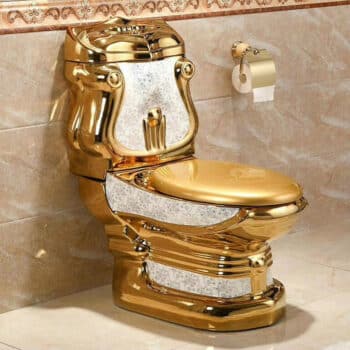This image showcases an extraordinarily ornate bathroom, featuring what must be one of the most lavish toilets ever seen. The toilet itself is predominantly golden, adorned with intricate white marbling that gives it a regal appearance, almost as if it were designed for royalty. The gleaming toilet is complemented by a gold lid, and a portion near the base showcases a black flowery pattern on a white background, adding to its lavish detail. 

The bathroom floor appears to be made of marble in a tan hue, while the walls have a peachy, marble-like finish, further enhancing the room's opulent aesthetic. Chair molding or decorative tile surrounds the area immediately around the toilet, contributing to its luxurious ambiance. 

Even the toilet paper holder is ornate, with golden embellishments giving the impression that the paper emerges from a gilded mount. Despite the extraordinary wealth on display, the bathroom also contains the familiar, everyday detail of plain white toilet paper, situated to the right of the toilet.

This extravagant display, while impressive, might also invoke thoughts of excess and decadence, making it a subject of both admiration and criticism. Overall, the scene is fit for a king or queen, illustrating a stark contrast between opulence and functionality.